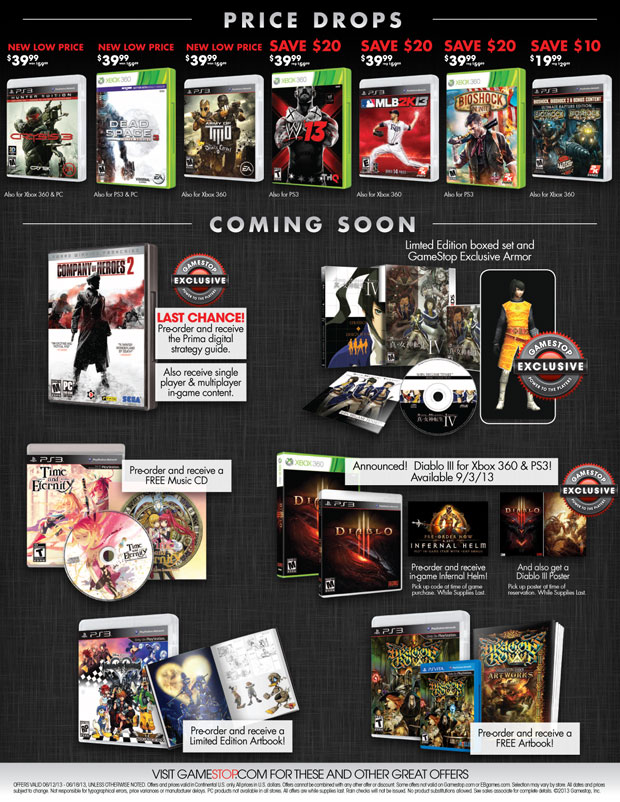This promotional image highlights a selection of seven video games, all prominently featuring their cover art and discounted prices. Each game is now available for $39.99, down from the original price of $59.99. A bold red text exclaims "New Low Price," with some titles also featuring a "Save $20" annotation. At the top of the image, "Price Drops" is written in striking silver text.

Below these discounted games, there is a "Coming Soon" section showcasing upcoming releases. The first game highlighted here is a GameStop exclusive, conveyed with a sign that reads, "Last Chance! Pre-order and receive the Prima Digital Strategy Guide." Additional incentives include both single-player and multiplayer in-game content, as well as a limited edition boxed set and exclusive armor for GameStop purchasers. The cover art displays a character dressed in a yellow outfit with gray sleeves.

Additionally, there is an opportunity to pre-order and receive a free music CD for a game named "Timik and Ursify," featuring two characters—one with blonde hair and the other with pink hair. Another notable announcement is for "Diablo 3," slated for release on Xbox 360 and PS3 on September 13, highlighted by "Announced: Diablo 3" text.

The image concludes with a call to action, inviting viewers to visit GameStop.com for these and other great offers, making it evident that the entire layout is designed as a promotional advertisement for GameStop.